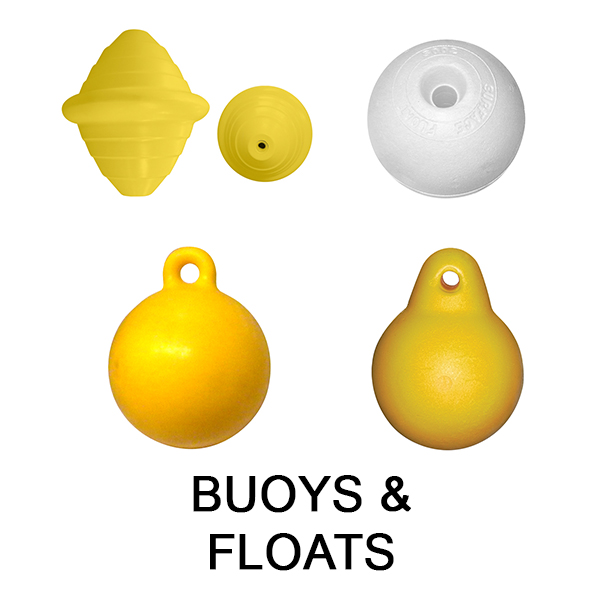This image, seemingly extracted from a professional website focused on marine equipment, prominently displays buoys and floats against a stark white background. The composition is divided into four quadrants, each showcasing a different buoy or float, all in various shades of yellow and white. 

In the top left quadrant, there is a yellow, diamond-shaped buoy with a ribbed texture, depicted both from the side and from a top view, where it appears as a circle with a central hole. Adjacent to it in the top right quadrant, a white spherical float can be found, featuring a hole at the top and faint engravings that are difficult to discern.

The bottom left quadrant houses another yellow buoy, resembling an orange with a handle, while the bottom right quadrant features a similarly shaped buoy, distinguished by its thicker handle walls. All objects are meticulously placed, each occupying their respective quarter of the image.

Centrally located at the bottom is the text "BUOYS FLOATS," set in a black, sans-serif, all-caps font. The professional nature of the image and its simplistic yet informative design suggest that it likely originates from a specialized website dedicated to marine buoys and floats.